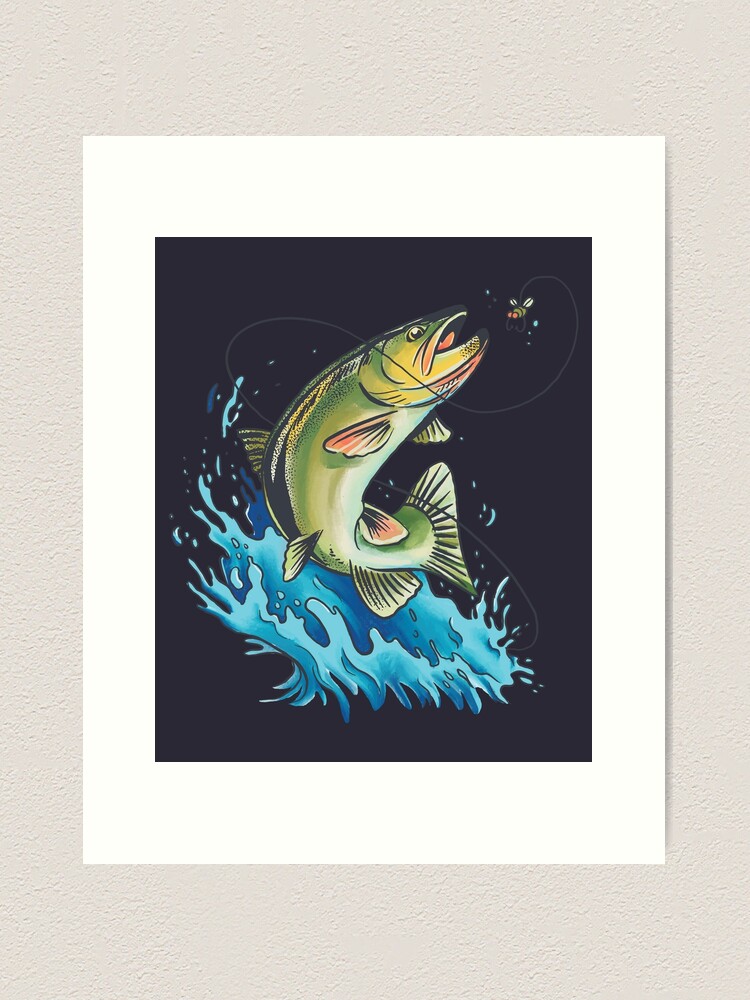The image showcases a detailed painting of a green and yellow fish, possibly a wide-mouth bass, as it leaps energetically out of splashing blue water. The fish has peach-colored fins with pink accents near its mouth, orange and green gills, and a dynamic mix of navy blue hues swirling around it. It is in hot pursuit of an insect, which dangles tantalizingly in front of its open mouth, tethered by a gray string that curls and snakes through the scene. The artwork is set against a solid black background and is enclosed within a wide white matte frame. This framed painting hangs on a textured beige wall, adding a striking visual contrast to the wall's subdued tones.